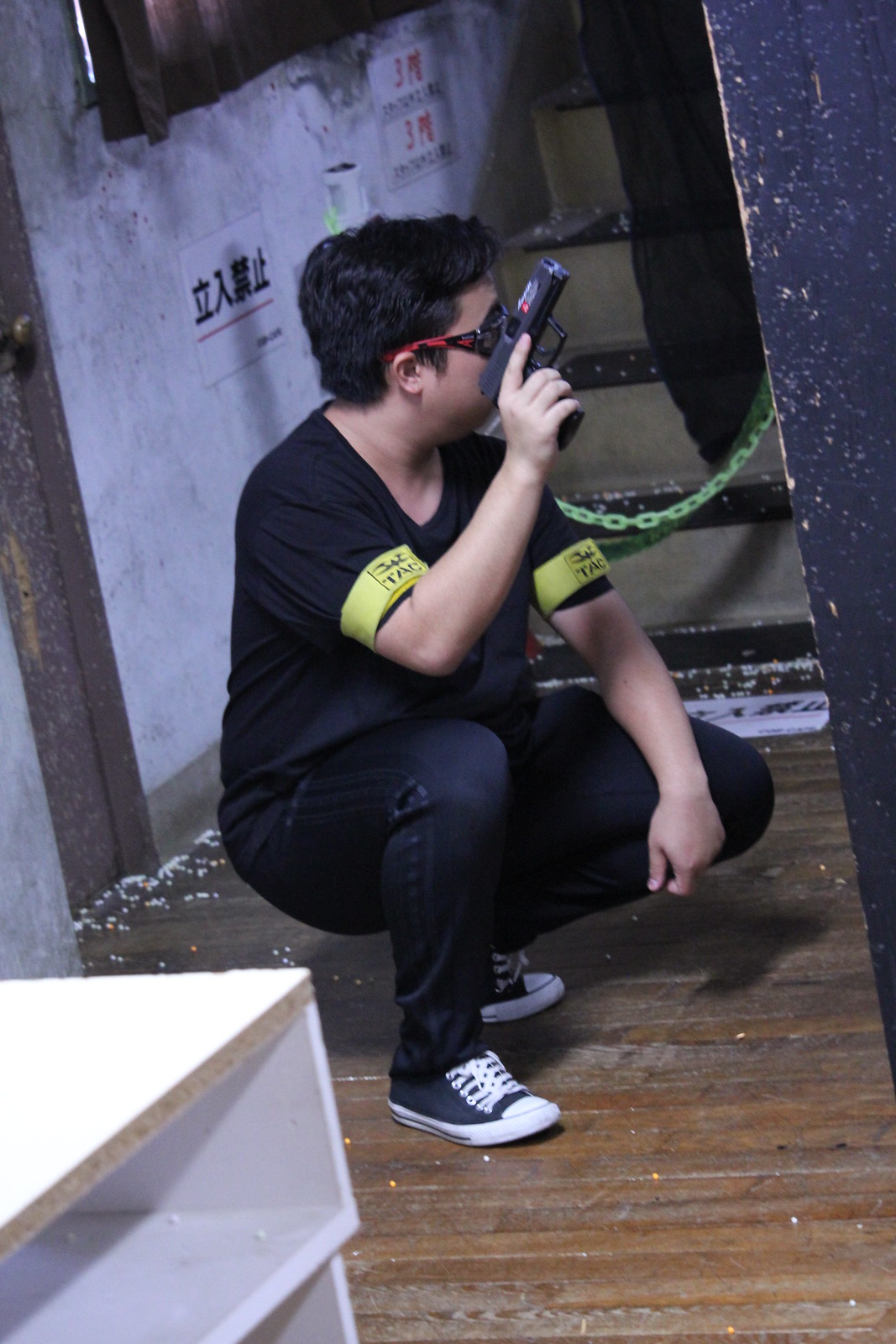The image vividly captures a man in a dynamic crouching position, reminiscent of participation in a laser tag game. He is adorned in black jeans, a black t-shirt, and black and white sneakers. Striking red-rimmed glasses frame his face, complemented by short black hair. Yellow bands emblazoned with "tag" grip tightly around his biceps, indicating his involvement in the game.

In his right hand, he wields a black toy laser gun, adding to the game's authenticity. The setting is an intriguing blend of old and new: an ancient building with wooden floors and white-painted walls stands in stark contrast to the modern elements of the game. A white drawer peeks from the bottom left corner, and a green chain cordons off an area leading to a flight of stairs. Signs adorned with Asian-style letters punctuate the bright, well-lit room, adding an exotic flair. The man, appearing unaware of the camera, exudes a sense of urgency and strategy, deep in the game's immersive experience.